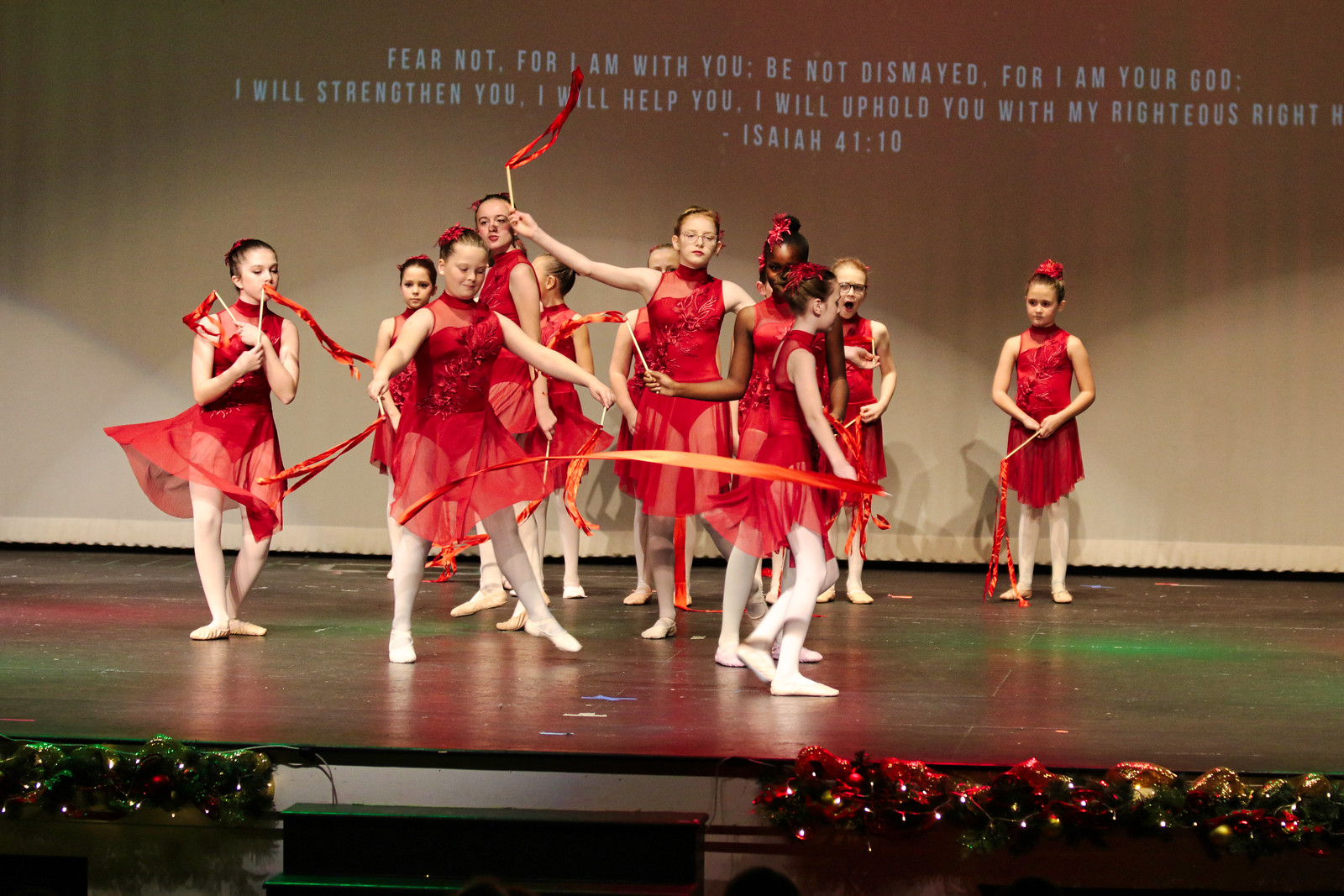This photograph captures a group of young girls, ranging in age from about 8 to 16, standing on a stage likely preparing for a dance performance. They are all dressed in deep Valentine-red ballet costumes, featuring sheer skirts and sheer panels near the neck, paired with white leggings and white ballet slippers. Red bows adorn their hair, adding to the coordinated appearance. Each girl is holding a stick with red ribbons attached, reminiscent of the props used in rhythmic gymnastics. The stage itself is dark brown, decorated with Christmas lights, plants, and possibly other festive elements which are not clearly discernible. The background features a beige curtain with a projection that reads in bold blue block letters: "Fear not, for I am with you. Be not dismayed, for I am your God. I will strengthen you. I will help you. I will uphold you with my righteous right hand." The reference to Isaiah 41:10 is also visible. The performers are in various states of readiness, some appearing a bit hesitant while others are starting to move, suggesting this might be a warm-up or practice session for an upcoming event.